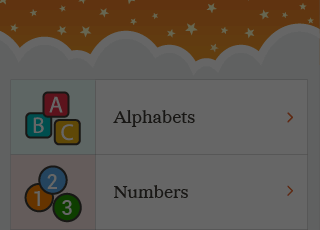This image is a low-quality, small square screenshot with a muted gray filter overlay. It features an orange background at the top, decorated with small white five-pointed stars. Below the orange section, a graphic of fluffy clouds is visible. 

Under the cloud graphic, there are two white rectangles containing icons and text on the left side. In the top rectangle, there is an icon depicting children's wooden blocks, each labeled with a letter and colored differently: the top block is 'A' in red with white font, the middle block is 'B' in blue with white font, and the bottom block is 'C' in yellow with white font. Next to the blocks, the word "Alphabets" is written in black font, accompanied by a small arrow pointing to the right.

The lower rectangle contains an icon of colored circles numbered 1, 2, and 3: the '1' is yellow, the '2' is blue, and the '3' is red. Adjacent to the circles, the word "Numbers" is displayed in black font.